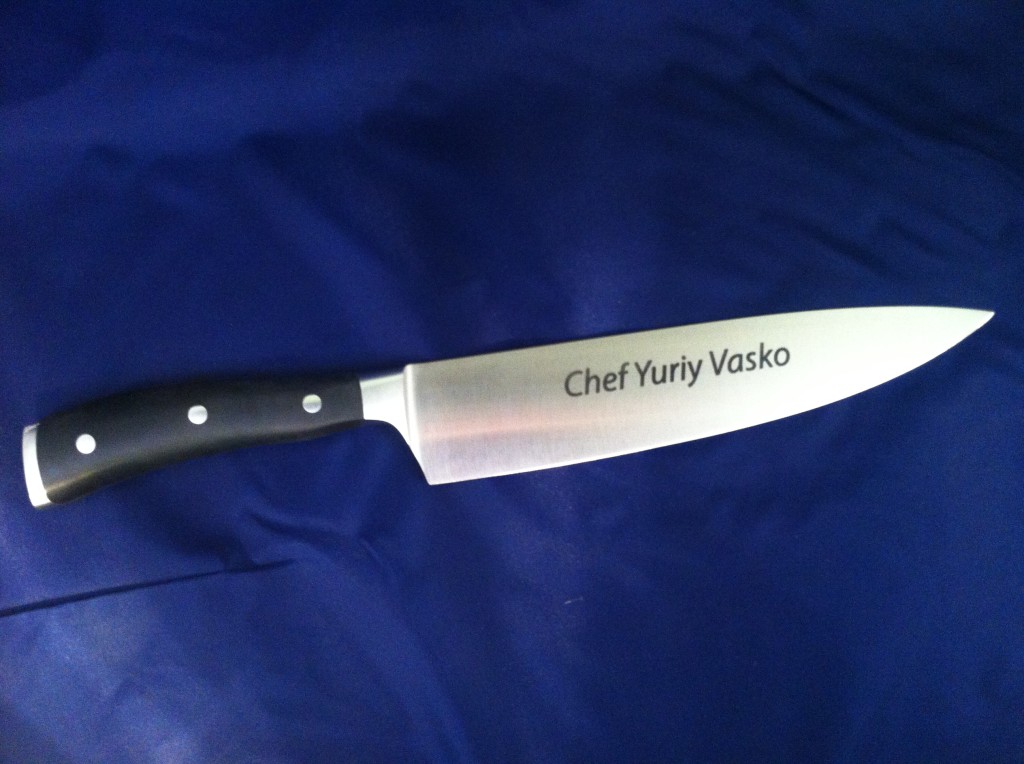The image features a high-quality chef’s knife prominently displayed against a dark blue, silky or velvety fabric that could be a tablecloth or blanket. The knife is oriented slightly diagonally but mainly vertical, with the handle at the top and the blade at the bottom. The handle is black and adorned with three silver pins, highlighting its sturdy build. The blade is a shiny, elegant silver, inscribed with the text "Chef Yuriy Vasko" along its length. The scene suggests a setting that could be either a bedroom or kitchen, possibly styled for an online store to showcase the knife, indicating it may be for sale. This personalized chef’s knife, with its distinctive, non-English name, underscores its intended use by a professional, emphasizing its high quality and importance in culinary tasks.